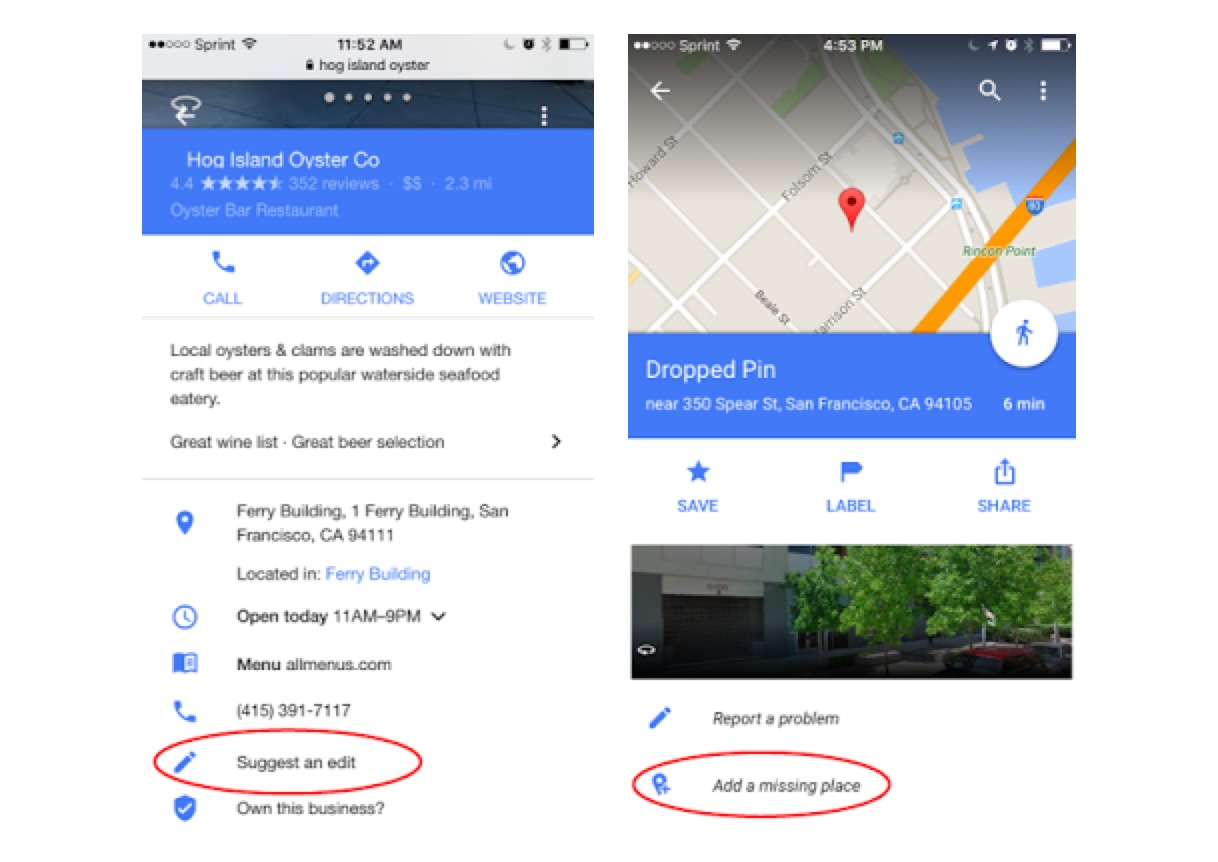In this image, there are two cell phone screenshots displayed side by side. 

**Left Screenshot Description:**
- At the top of the left screenshot, there is a gray status bar with several icons including a battery icon, Bluetooth icon, clock icon, "Do Not Disturb" icon, and Wi-Fi icon. The time is shown as 11:52 AM.
- Below the status bar, the text "sprint" is written on the screen, with a locked padlock icon displayed near the text "Hog Island Sister."
- A section title, "Hog Island Oyster Co.," is displayed below the gray bar in white text over a blue background.
- Beneath the title, there are blue hyperlinked options: "Call," "Directions," and "Website."
- The description of the place reads: "Local oysters and clams are washed down with cash beer at the popular obsessive food eatery. There's a great wine list and a great beer selection." This text appears in black ink.
- Various details about the location, such as the operational hours, menu, and contact number, are presented.
- Certain parts of the text are circled in red, with labels such as "Suggest an edit" and "Own this business."

**Right Screenshot Description:**
- The right screenshot displays a continuation of the information from the left screenshot but includes a map highlighting the location of Hog Island Oyster Co.
- The drop pin for the place is shown, along with options to "Save," "Label," or "Share" the location.
- The image also includes a picture of the venue.
- Additional text options are available, such as "Report a problem" and a red-circled prompt to "Add a missing place."

These screenshots provide a comprehensive overview of the Hog Island Oyster Co., including contact details, operational hours, map location, and additional options for user interaction and reporting issues.